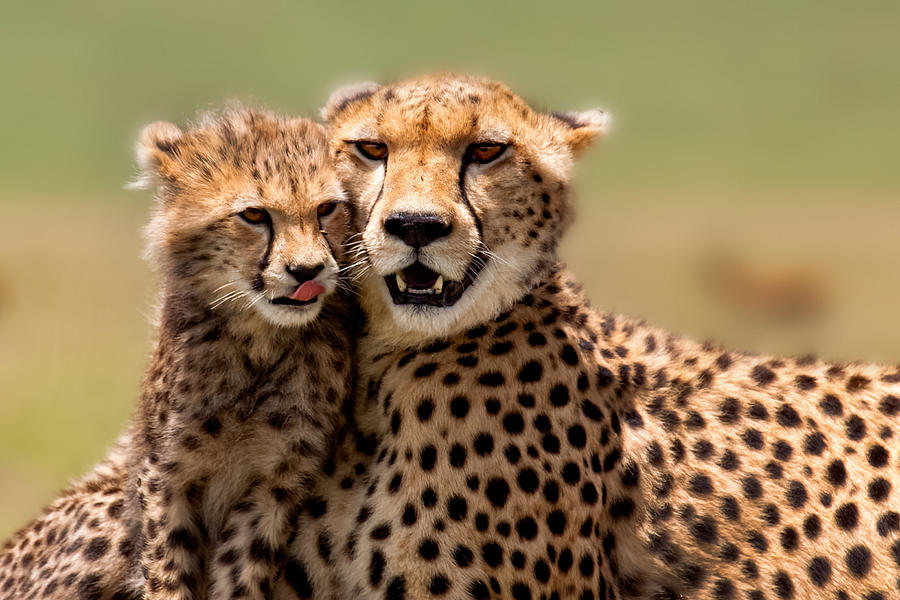In this color photograph taken in daylight, a mother cheetah and her cub are lovingly nestled against each other in an open area. The cub, positioned on the left, is cuddling up to its mother, leaning on her for comfort with its tongue sticking out as it licks its black nose. The mother cheetah, to the right, appears to be panting, with her mouth slightly open, revealing her lower fangs and teeth. Both cheetahs possess golden fur adorned with dark brown spots, and distinctive black tear lines that run from their eyes to their mouths. Their heads are tenderly pressed together, capturing a moment of closeness. The well-lit scene shows their shadows cast directly downward, indicating the sun is high above. The background is a blurred mix of green grass and patches of brown dirt, emphasizing the subjects in the foreground.